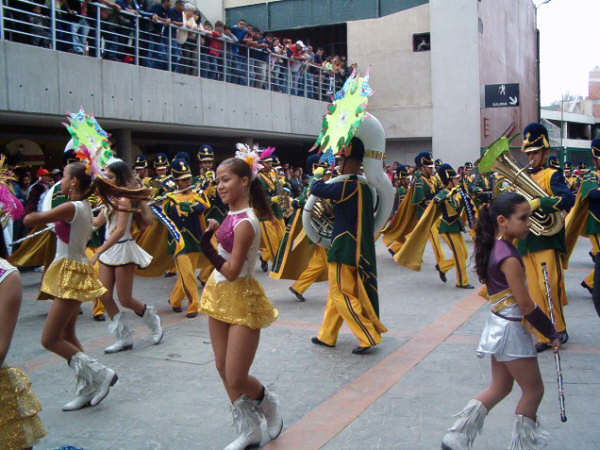The image depicts a vibrant scene of a marching band performance taking place outdoors in what appears to be a high school or sports stadium parking garage. The band members are clad in identical uniforms featuring blue and green jackets with gold trim, complemented by gold yellow pants with black stripes down the sides. Many members sport elaborate tall hats with gold tassels, and some wear capes. They are playing a variety of instruments, including tubas, trombones, and flutes, creating a lively atmosphere in the daylight.

Adjacent to the band, cheerleaders and baton twirlers, likely part of a flag team, are energetically performing dance routines. The cheerleaders are dressed in white shirts with pink accents and gold skirts, accessorized with white boots adorned with fringe. Their hair is styled in ponytails, adding to the coordinated and polished look of the group.

To the left of the performers, a raised balcony area with a railing holds a crowd of onlookers who are eagerly watching the performance from above, suggesting that this is a multi-level structure with spectators viewing from what seems to be an upper level or parking garage. The background hints at a stadium environment with visible seating areas, while the sky is overcast, providing a diffuse white backdrop to the scene. The overall atmosphere is one of excitement and celebration as the large marching band and cheerleading squad deliver their dynamic performance.